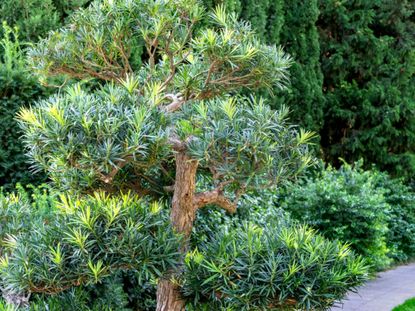This photograph, taken outdoors, captures a small cedar tree with rugged brown bark and needle-like green leaves. The cedar appears shrubbish, with compact branches in varying shades of green, darker at the center and more lime-green towards the tips. The tree exhibits a unique twisted growth with layers of foliage separated by segments of the trunk. Surrounding the cedar are additional shrubs with similar needle-like leaves. In the background, tall arborvitae trees stand prominently, characterized by their closely packed, green leaves that grow in a cylindrical, torpedo-like shape. To the right, we see larger, older pine trees and other dense bushes. A small section of a gray paved walkway and a patch of grass are visible in the bottom right corner, adding to the natural ambiance of the scene.